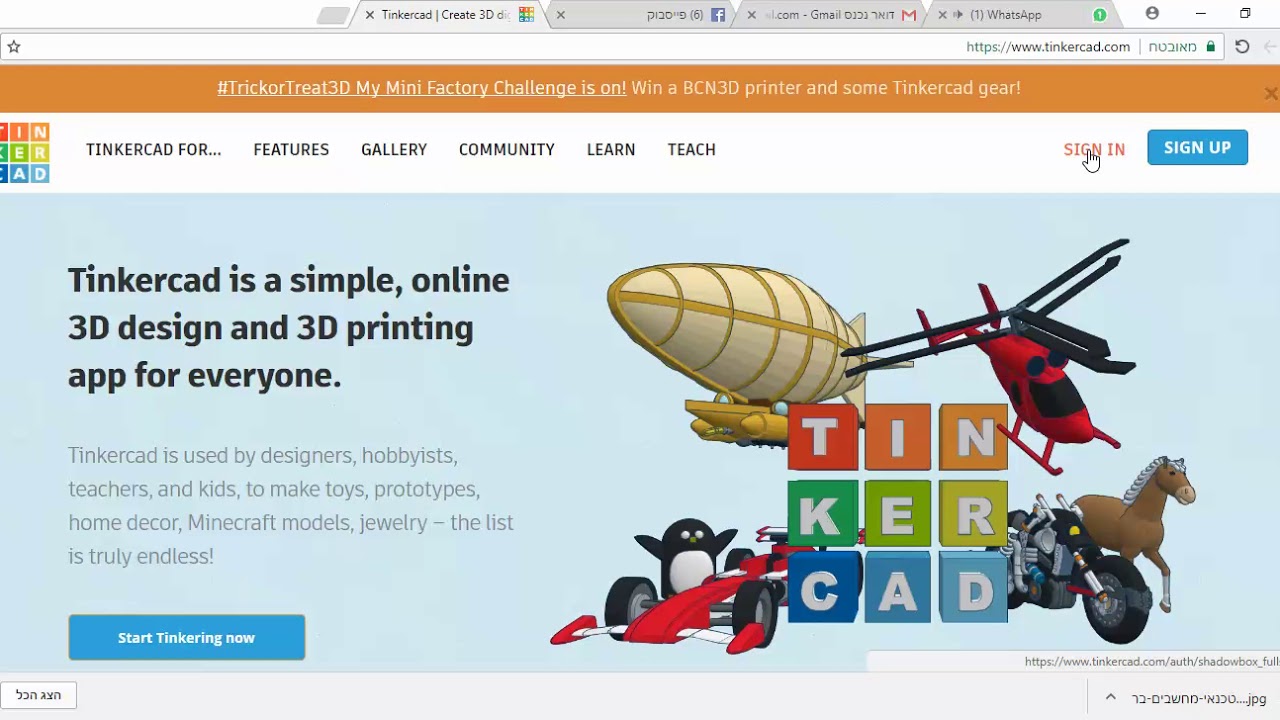This image showcases the homepage of Tinkercad.com, displayed in a web browser. The primary focus of the page is an illustrated scene of multicolored building blocks arranged in three rows. Each block contains a letter, with the first row spelling out "T I N," the second row "K E R," and the third row "C A D." 

Surrounding the blocks are whimsical, cartoon-style illustrations of a hot air balloon, helicopter, motorcycle, horse, sports car, and a penguin. These elements add a playful touch to the scene.

To the left of the blocks, there is text reading "Tinkercad is a simple online 3D design and 3D printing app for everyone." A blue button with white text is located at the bottom left corner of the page, reading "Start Tinkering Now.”